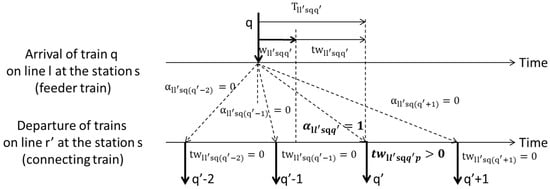This image showcases a detailed mathematical formula set against a white background, with all text and symbols in black. At the top left, the image features two neatly spaced-out paragraphs. The first paragraph reads, "Arrival of train Q on line 1 at stations (feeder train)." Directly below, the second paragraph states, "Departure of trains on line R at the stations (connecting train)."

The center of the image is dominated by a series of complex algebraic equations. The first equation starts with "T11SQQ," followed by an arrow guiding to the right, labeled "time." Below and interconnected with dotted lines are further equations, like "nSQ(Q-2) = 0." These equations cascade downwards, aligning with the text about the departure of trains. Midway through, a significant horizontal line is marked "time = 0."

The bottom of the image culminates with equations detailing variables such as "Q-2, Q-1, Q, and Q+1," illustrating a sequence of calculations. Arrows navigate back and forth among these equations, representing their interdependent relationships in time and space regarding the trains' schedules and mathematical modeling.